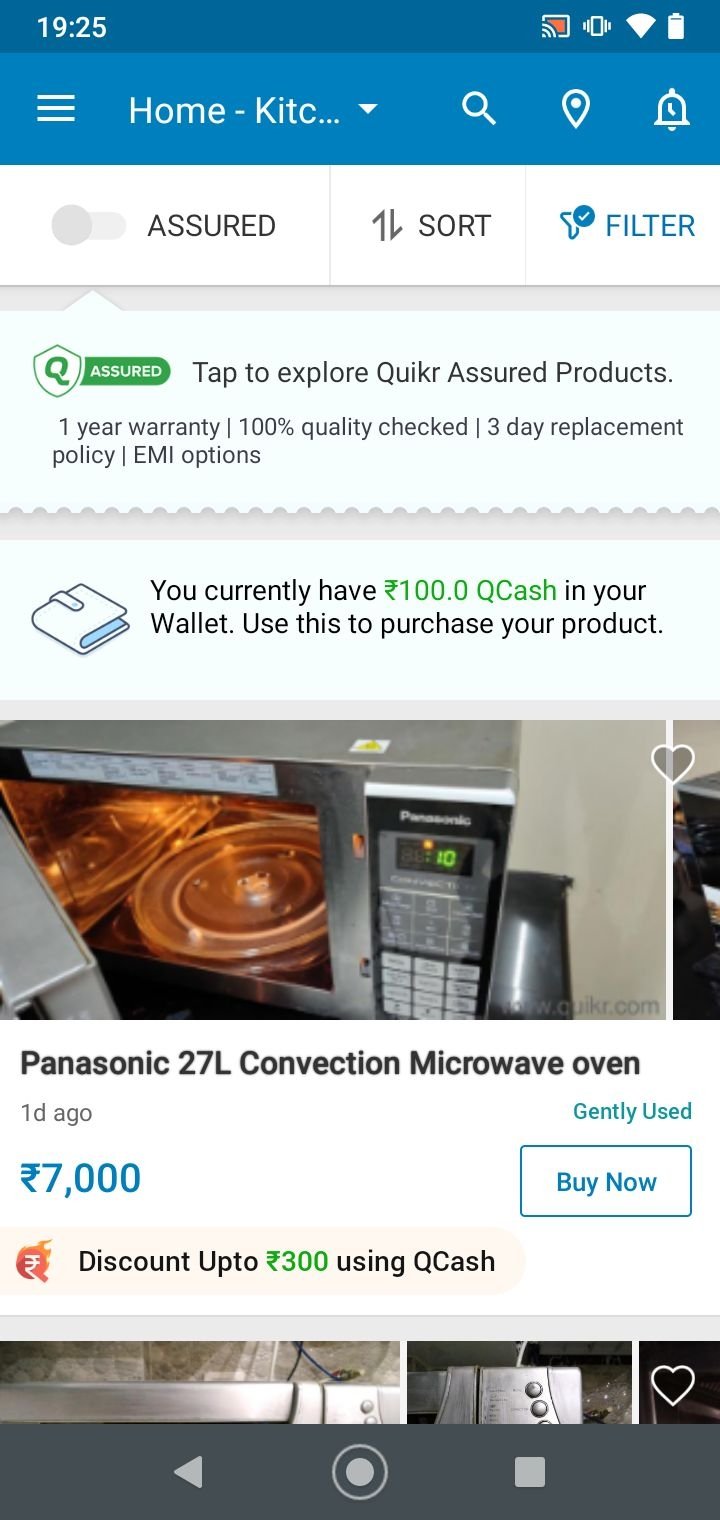A detailed cell phone screenshot description:

At the top of the screenshot, the current time is displayed on the left side, while various icons are clustered on the right. Just below this, a navigation bar features a blue rectangle on the left with three lines indicating a menu button. To the right of this menu button, there are several icons and text: "Home," "K-I-T-C," followed by three dots, a filled-in V-shaped down arrow, a magnifying glass, a location icon, and a bell.

Below the navigation bar, there's a toggle switch labeled "Assured," followed by the text "7L sort." Adjacent to this, there’s a filter icon with the word "Filter" displayed in blue. 

Further down, a prominent blue rectangle with the text "Tap to explore, Q-U-I-K-R Assured Products" catches the eye. Supplementary information within this section includes assurances such as a one-year warranty, 100% quality check, a three-day replacement policy, and EMI options.

Another light blue rectangle follows, announcing in green text: "You currently have $100 cash in your wallet. Use this to purchase your product."

Lastly, an image of a microwave is presented. The microwave is silver with its door open. Below this image, the product name is boldly stated in black: "Panasonic 27L Convection Microwave Oven." The product is available for purchase with a price tag of 7,000 pounds, accompanied by a "Buy Now" option.